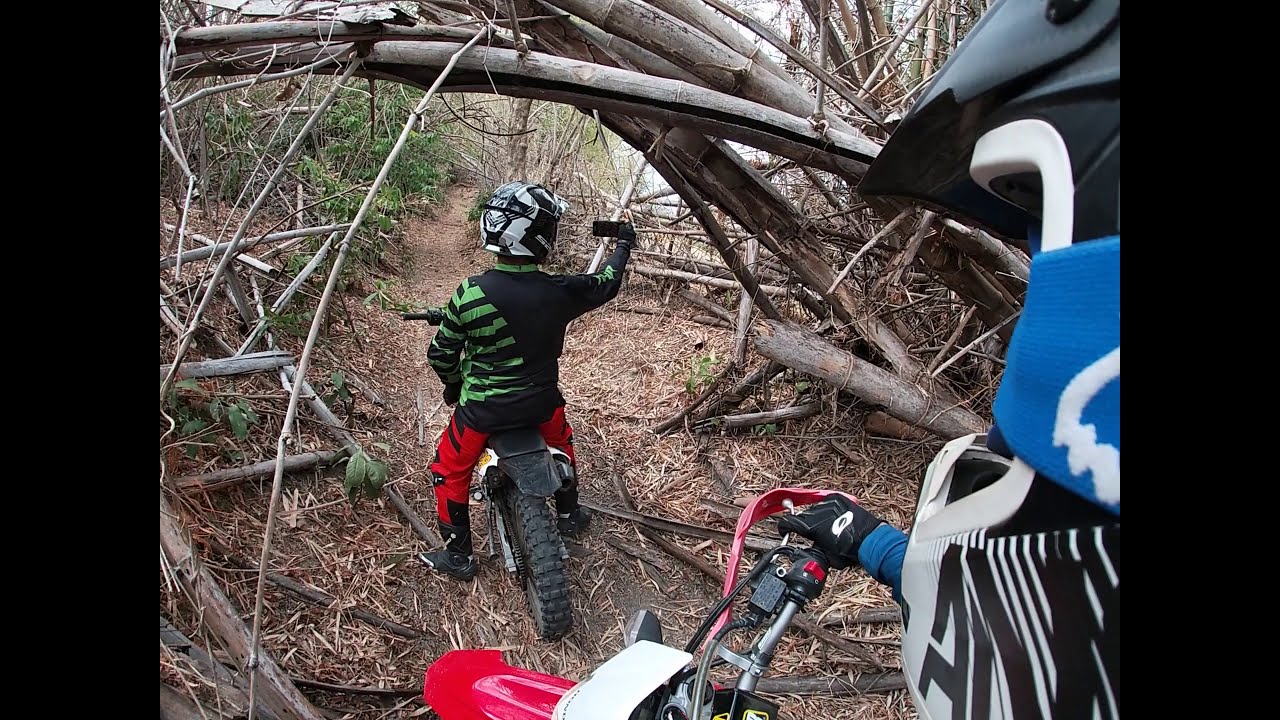In this photograph, we see two young children on small dirt bikes taking a break on a narrow forest trail. The trail is covered in fallen pine needles and complemented by small bushes on the sides. The children are about to pass under a natural tunnel formed by fallen, ancient trees with grayish-brown trunks. One child, wearing red pants, a green and black striped shirt, and a gray and black helmet, is in the lead and seems to be poking at the overhanging trees with a stick, expressing curiosity. The second child, closest to us, is on a red and white dirt bike and wearing a black, white, and blue helmet. This child appears to be taking a selfie with a cell phone, possibly using a helmet camera to capture the moment from their perspective. The picture poignantly captures a brief halt in their woodland adventure, emphasizing their youthful exploration and the enchanting forest setting.